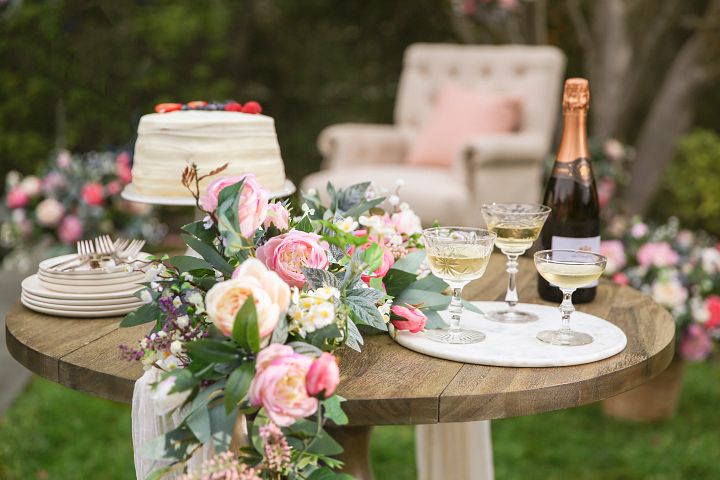The photograph captures an outdoor daytime scene, likely from a wedding or bridal shower. The focal point is a light brown round wooden table set amidst a garden. On the right side of the table, there is an unopened bottle of champagne with a gold foil top, accompanied by three champagne-filled crystal glasses arranged on a round white tray. The centerpiece of the table features a lush floral arrangement with light pink and yellowish roses, interspersed with green leaves, cascading over the table's edge. To the left, there is a stack of white plates with forks, and adjacent to it, a lavish, uncut layer cake topped with fresh strawberries and blueberries. The background is slightly blurry, showcasing additional potted flowers and a comfortable chair, enhancing the charming garden ambiance.